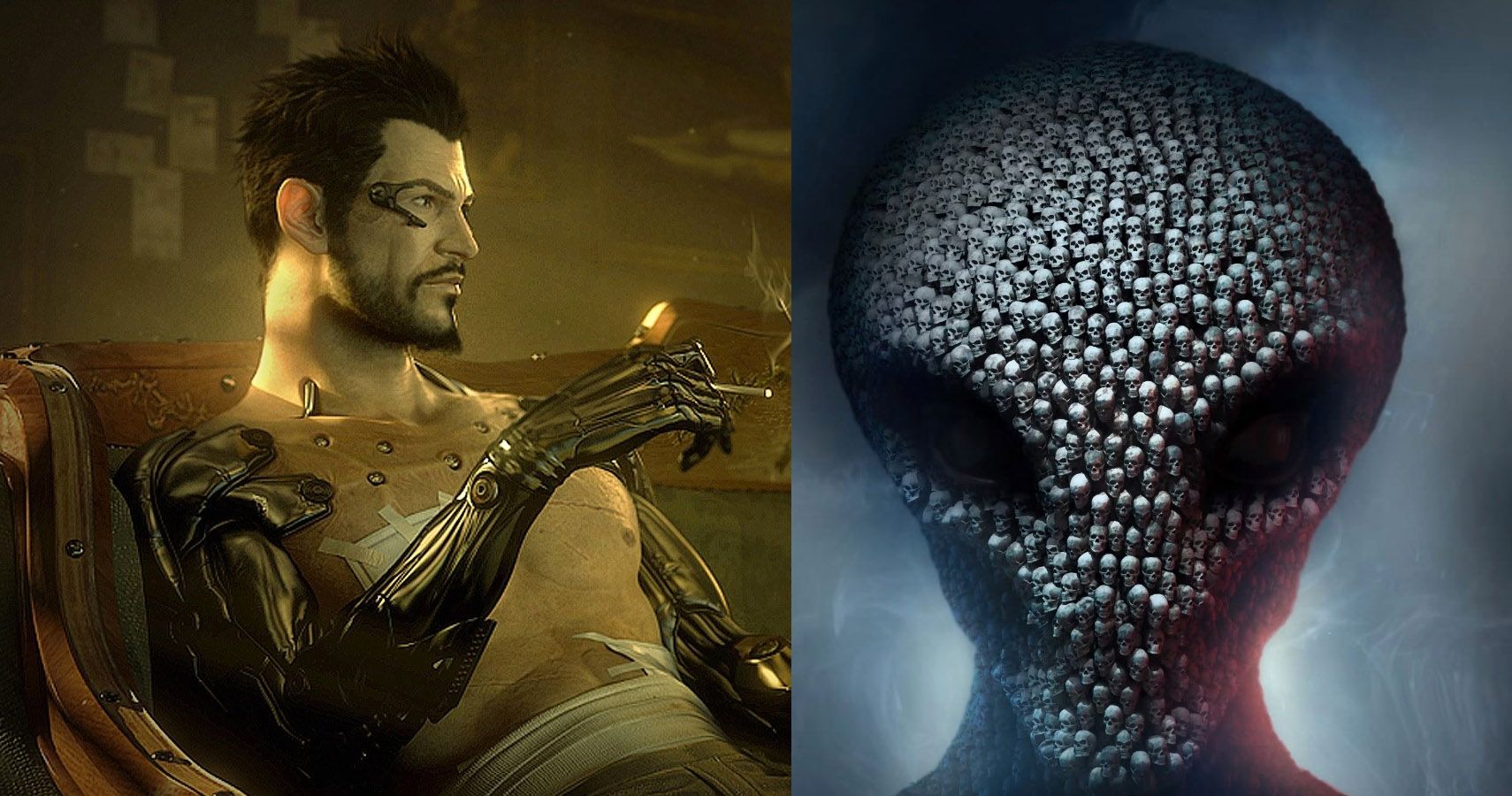The image is a composite split into two side-by-side sections, showcasing computer-generated art. On the left, an adult male with short hair, a pointed goatee, and a thin mustache leans back casually in a wooden chair. He is adorned with bionic, metallic arms and has a device implanted into his right temple. A bandage covers his waist and parts of his right chest, suggesting injury. The lighting casts a golden hue, lending an almost archaic atmosphere to the scene. In his right hand, he holds a cigarette, gazing off into the distance. The right side features an alien face with a pointed chin, large dark eyes, and a rounded forehead. The alien’s visage is intriguingly pieced together from an assemblage of human skulls, which create a haunting texture. The skulls are brighter at the top, contributing to a distinct, eerie light contrast against the gray background.